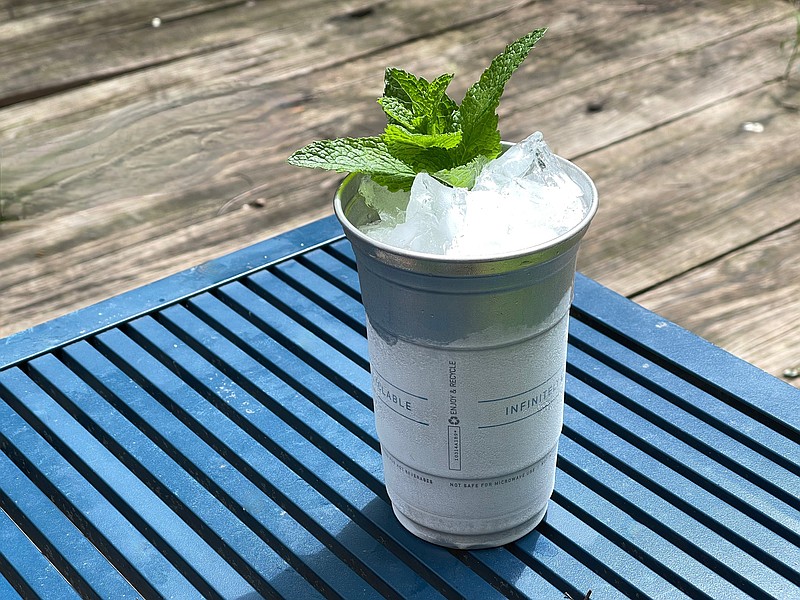This photograph features a close-up of a distinctive drink, likely a mint julep, placed prominently at the center of the image. The drink is served in a metal cup adorned with condensation and frost, indicative of its cold temperature. The cup is predominantly white with a blue rim and seems to have some text on it, though the writing is blurry and difficult to read. At the top of the cup, green mint leaves garnish the icy, clear liquid inside, enhancing the refreshing and citrusy appearance of the beverage.

The setting suggests an outdoor cafe environment. The cup sits on a reflective metal table, which rests on a wooden porch with visible slats. In the background, portions of a gray picnic table are visible on both the left and right edges of the image. The overall color palette includes shades of green from the mint leaves, the translucent white of the ice, the blue accent on the cup, the gray of the picnic table, and the brown tones of the wooden surface beneath it all, creating a cozy and inviting outdoor ambiance.